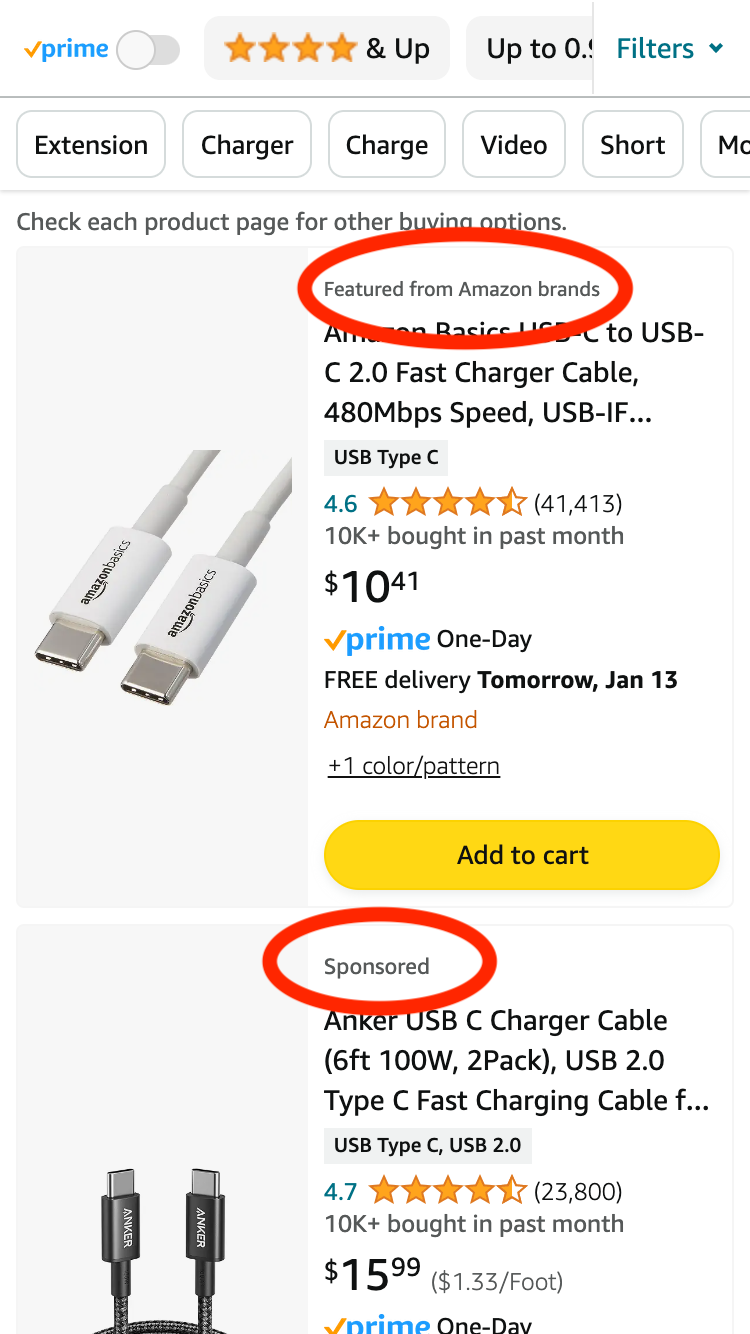**Detailed Caption:**

This screenshot, set against a white background, showcases an Amazon product page featuring multiple elements of interest. At the top, there is a rating of 4.6 stars based on 41,413 reviews. The main product highlighted appears to be a USB-C to USB-C 2.0 fast charger cable from the Amazon Basics line, partially cut off in the image. The cable is advertised with a data transfer speed of 480 Mbps. 

A notable feature is the price, listed at $10.41, and the product is marked with a check indicating Prime One-Day availability, promising free delivery by January 13th. Additionally, there is a yellow oval button suggesting to "Add to Cart." 

In the center of the screenshot, a red circle emphasizes the "Featured from Amazon brands" label, informing potential buyers about alternative products. The word “Sponsored” is also circled in red, suggesting that this particular item might be a promoted listing.

Towards the bottom, there is another highlighted product, an Anker USB-C charger cable, noted for its 6-foot length and 100W power capacity. This product is marketed as a 2-pack USB 2.0 type C fast charging cable.

Overall, this detailed view provides a snapshot of various shopping options and specific features, which include compatibility, performance, and delivery benefits for Amazon shoppers.